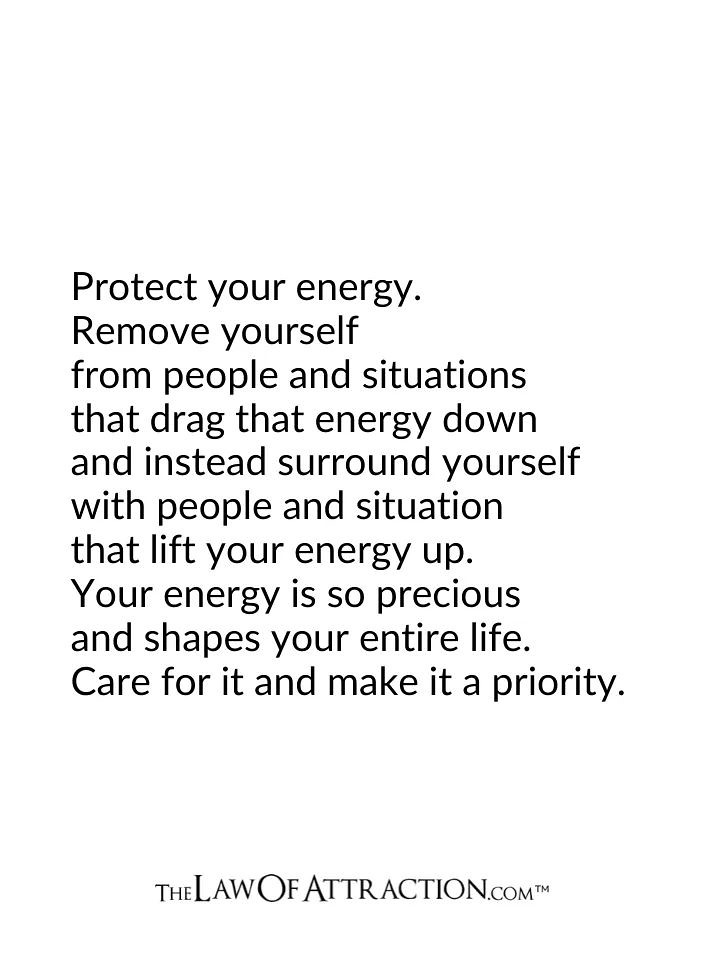The image features a simple yet impactful inspirational quote set against a plain white background, with clean, centered black sans-serif text. The message reads: "Protect your energy. Remove yourself from people and situations that drag that energy down, and instead surround yourself with people and situations that lift your energy up. Your energy is so precious and shapes your entire life. Care for it and make it a priority." The attribution at the bottom displays "thelawofattraction.com" in varying font sizes, with "the" and ".com" in smaller text and "law of attraction" in larger text, accompanied by a trademark symbol. This versatile graphic could adorn a card, a wall, social media feeds, or serve as a computer screen backdrop, reminding viewers to prioritize and cherish their energy in everyday life.